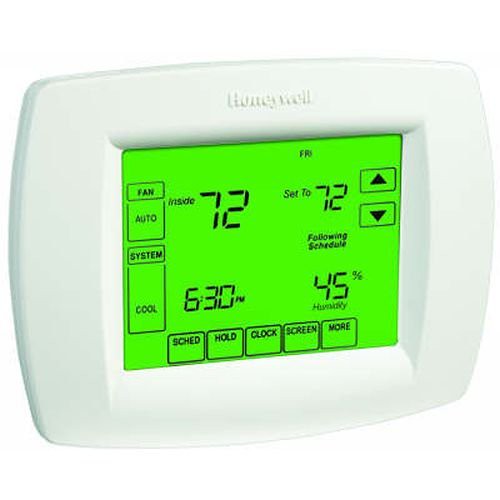This image features a real-life Honeywell appliance LED control panel, likely from an HVAC system such as an air conditioner. The panel is photographed against a white background, enhancing its distinct design. The panel itself is encased in a thick, curved rectangular border. Within this frame is a smaller, rectangular LED screen with green backlighting, displaying black text and information.

On the left side of the screen, there are four distinct rectangular sections displaying the following text in all capital letters:
1. FAN
2. AUTO
3. SYSTEM
4. COOL

Along the bottom of the LED screen are five labeled boxes:
1. SKEDGE
2. HOLD
3. CLOCK
4. SCREEN
5. MORE

On the right side of the screen, two arrow buttons—represented by triangles pointing up and down—are housed within their own rectangular sections, presumably for adjusting settings.

In the center of the LED display, starting from the top left and moving outward, the following information is shown:
- The number "72" indicating the current temperature.
- To the right, the text "INSIDE" and further right, "SET 72".
- Below, the text "FOLLOWING SCHEDULE".
- Underneath, "45%" indicating humidity.
- Towards the top right, the time "6:30 PM".
- Adjacent to the time, the day "FRI" (Friday).

At the top of the plastic panel encasing the LED screen, the brand name "HONEYWELL" is embossed, marking its identity. The panel is meticulously crafted, blending functionality with a clear, user-friendly interface.